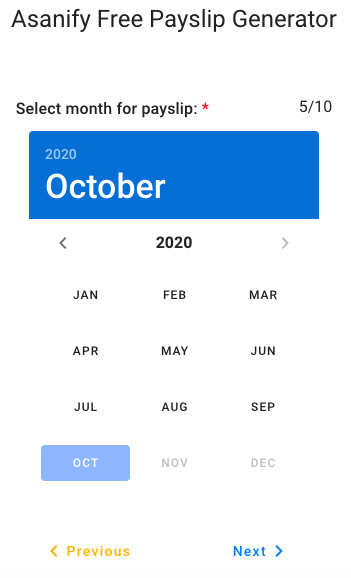This image displays the Sonify Free Payslip Generator interface for selecting a month. The interface is focused on the month of October 2020. The selection area prominently features a long blue rectangle with the month "October" written in white, highlighting it against the blue background. Below, a calendar section shows the entire year 2020. 

Each month is abbreviated from January (Jan) to December (Dec). The months from January to September are in bold black text, while October is highlighted with a shaded blue background. November and December are grayed out, indicating they are not currently selected. 

Additionally, there are navigation options at the bottom: "Previous" in orange with a left-pointing arrow, and "Next" in blue with a right-pointing arrow, allowing users to navigate between months. A red asterisk is also seen, indicating a required selection field. The overall design is clean and functional, emphasizing user interaction with the month selection feature.